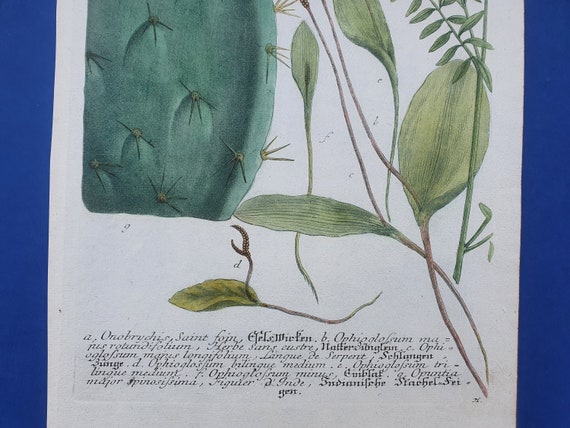The image depicts a white page, possibly from a textbook or slide, set against a blue background with blue borders running along the right and left sides. On this page, there are detailed illustrations of two plants. The plant on the left resembles a cactus, with a dark green stump covered with light green spikes. The plant on the right features long, thin green leaves attached to green stems, some of which resemble spoons. Below these illustrations, there is cursive text in a different language or possibly old English, which is difficult to decipher. The text provides names and descriptions of the plants, including terms like "Honor Bridges," "St. Foyne," and "Ophiogolium MA."